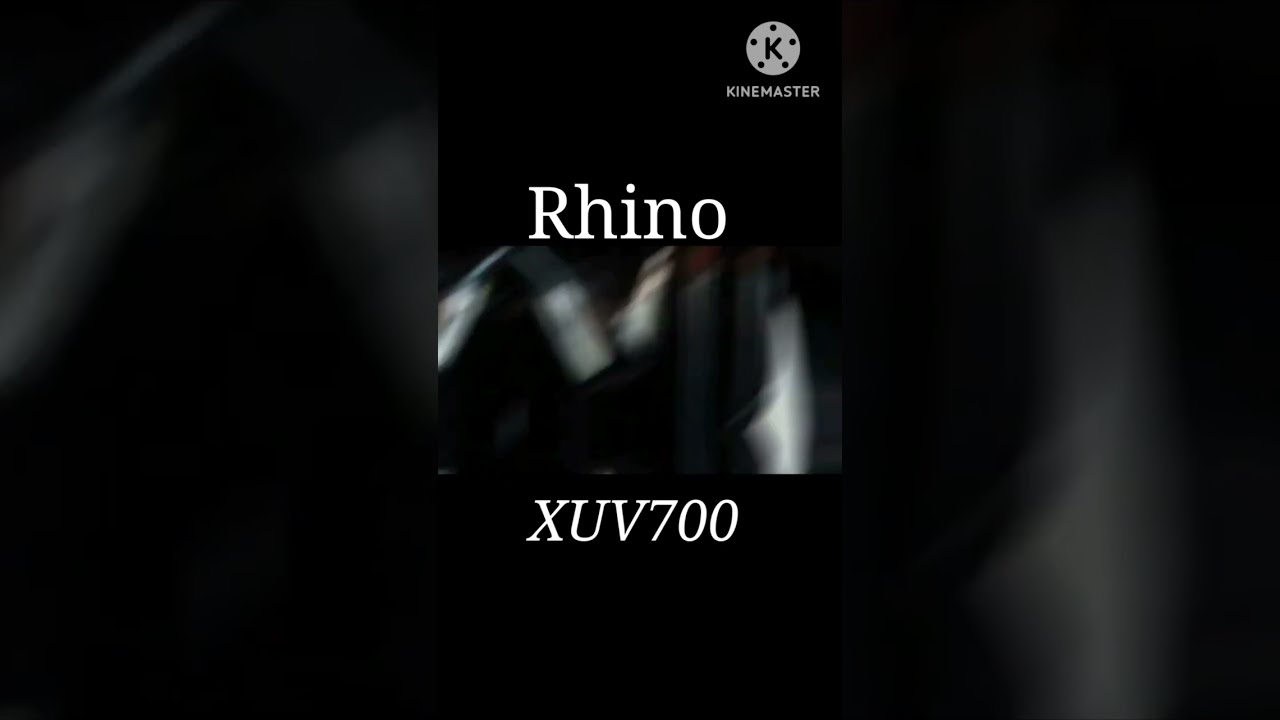The screenshot from the video features a predominantly black and gray background, with a blurry image in the middle that could possibly depict kneeling figures or a vague hand, making it difficult to discern the exact subject. In the upper middle section of the image, the word "Rhino" appears in white serif font, and below it, the text "XUV700" is italicized. Positioned in the top right corner is the KineMaster logo, consisting of a gray circle with five black dots surrounding a capital "K." This layout implies the screenshot may be related to video editing software or an advertisement. The faint colors and vague shapes present throughout the image add to the overall ambiguous and indistinct visual presentation.